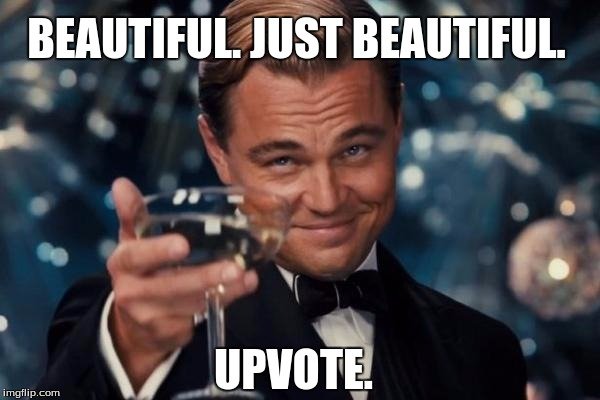The meme features actor Leonardo DiCaprio, possibly from "The Wolf of Wall Street" or "The Great Gatsby," dressed in a black tuxedo with a white button-up shirt and a black bow tie. He is slicking back his hair and grinning, his head slightly bowed as he raises a glass of champagne in a toast-like gesture. The background has a bluish hue with blurry, glittery elements, including what appears to be a disco ball or silver and blue balloons, indicating a festive and glitzy party scene.

At the top of the image, large white block letters with a black outline spell out, "BEAUTIFUL. JUST BEAUTIFUL." Similarly styled text at the bottom reads, "UPVOTE." In the bottom left corner, the small text, "imgflip.com," is visible in white. The overall ambiance of the image evokes celebration and class, with DiCaprio at the center of the toast.